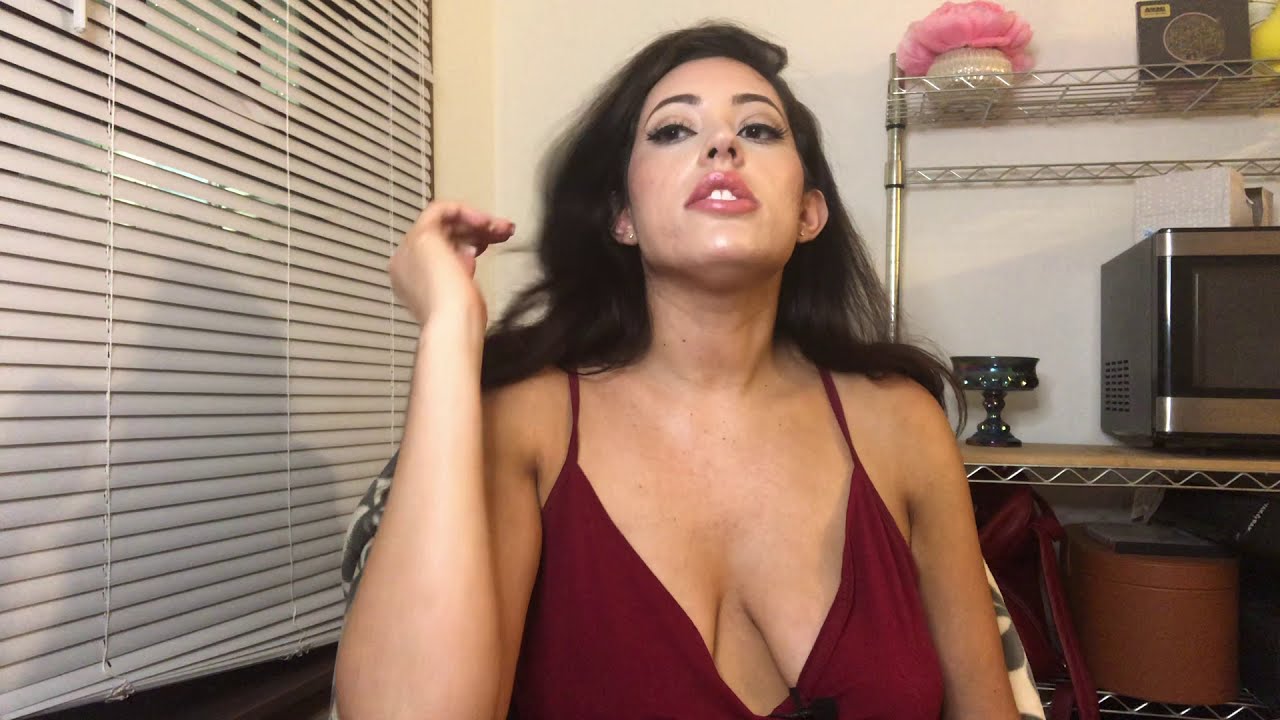The photograph captures a woman seated in what appears to be a kitchen or dining room area. Behind her stands a baker's rack housing various items: a microwave partially out of view on the right with a vase, a box, and a yellow object above it, and a candy dish to the left. Below these, there's a round, brown box and a red satchel. The room's backdrop is a plain white wall, and to the left of the woman, there are white blinds. The woman has shoulder-length brown hair parted to the side, brown eyes, and she’s wearing small stud earrings and a burgundy V-neck tank top. She is mid-motion, possibly taking a photo of herself with her right hand up near her face, which is slightly out of focus. Her chin is angled upward, and her lips are slightly parted, revealing her teeth.